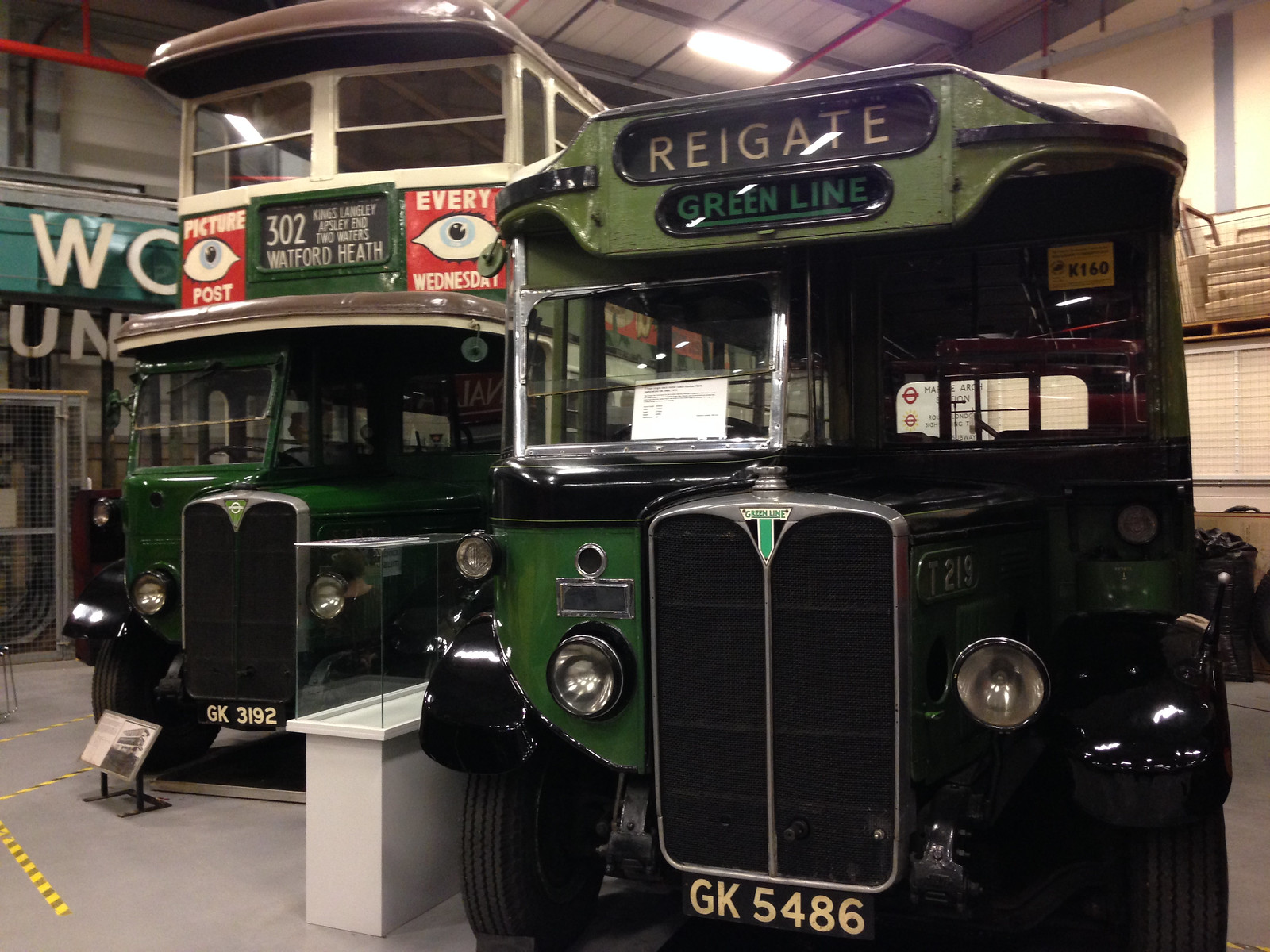This photograph showcases a collection of vintage buses displayed inside what appears to be a museum or a showroom. On the left, there is a double-decker bus with a green lower section and white upper section. This bus features multiple windows and some banners on its front, and its license plate reads GK3192, with a sign indicating "302 Watford Health" on the top side. To the right of this double-decker is a single-decker, army green bus. The license plate of this bus is GK5486, and the signage on its top reads "Regate Green Line". The single-decker bus also has two lit headlights and a bumper that appears different from modern buses. Both buses are distinctly old-fashioned and preserved well for display in this indoor environment.